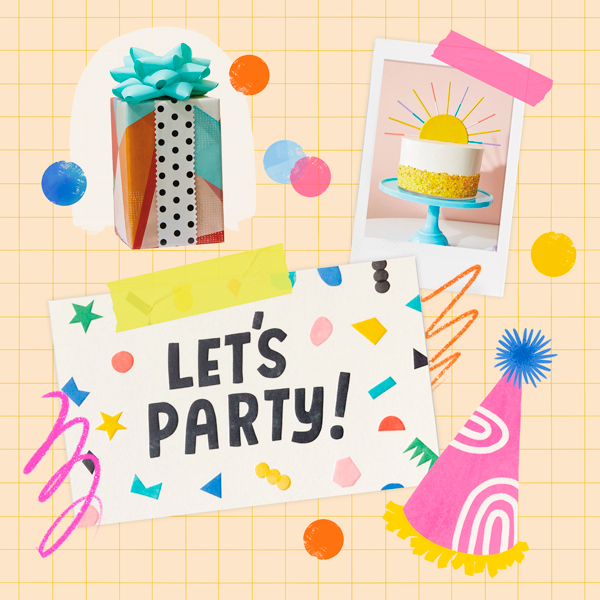This vibrant and cheerful birthday party invitation features a colorful collage on a checkered gold background. Central to the design are several lively images: a multicolored gift box adorned with a big, beautiful green bow and colorful balls around it; a Polaroid picture taped on, showcasing a white cake with a yellow crumb bottom and a decorative sun on top; and a spirited "Let's Party!" sign with confetti. Additionally, there's a pink party hat with white designs and a light blue pom pom ball. The collage is filled with various shapes like stars, triangles, and circles, and all elements together create an inviting and festive atmosphere.